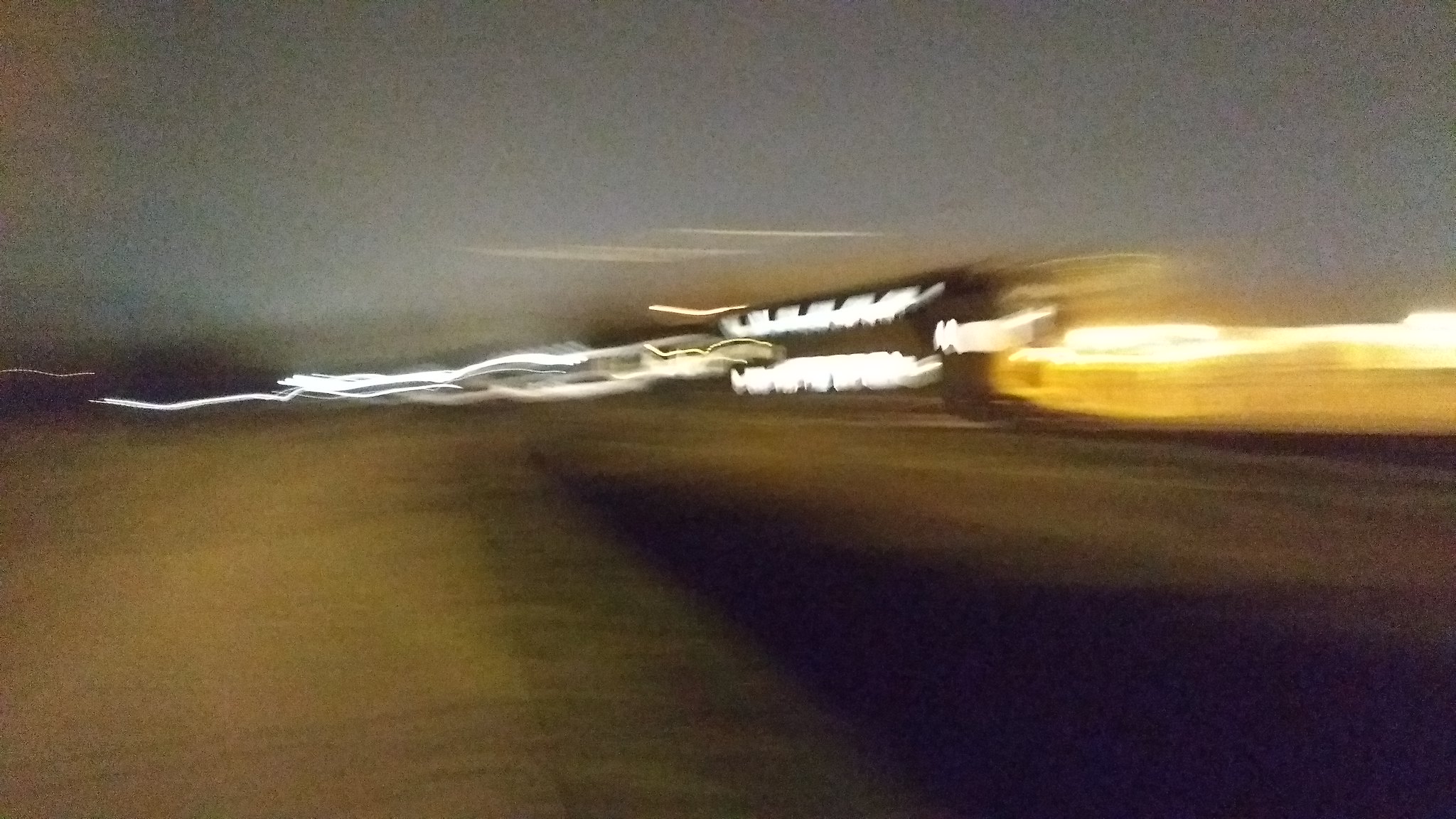An extremely blurry and distorted image depicting a scene that is difficult to decipher. Dominating the center of the image is what appears to be a building with lights on both levels, though its details are obscured. The lower half of the image shifts from a tan brown hue on the left to almost black in the middle, with a dark line ascending from the lower right to the left, potentially illustrating a roadway. On the left side, a series of ice blue and white light streaks suggest the movement of cars, typical of a time-lapse photograph. The right side of the image is bathed in a yellowish glow, hinting at early morning light, possibly from the rising sun. In the background, the sky is a faint gray-blue, giving the impression of an overcast evening or almost nighttime, with blurred clouds passing in the foreground. There might also be a small tower with lights on, positioned to the right of the building.